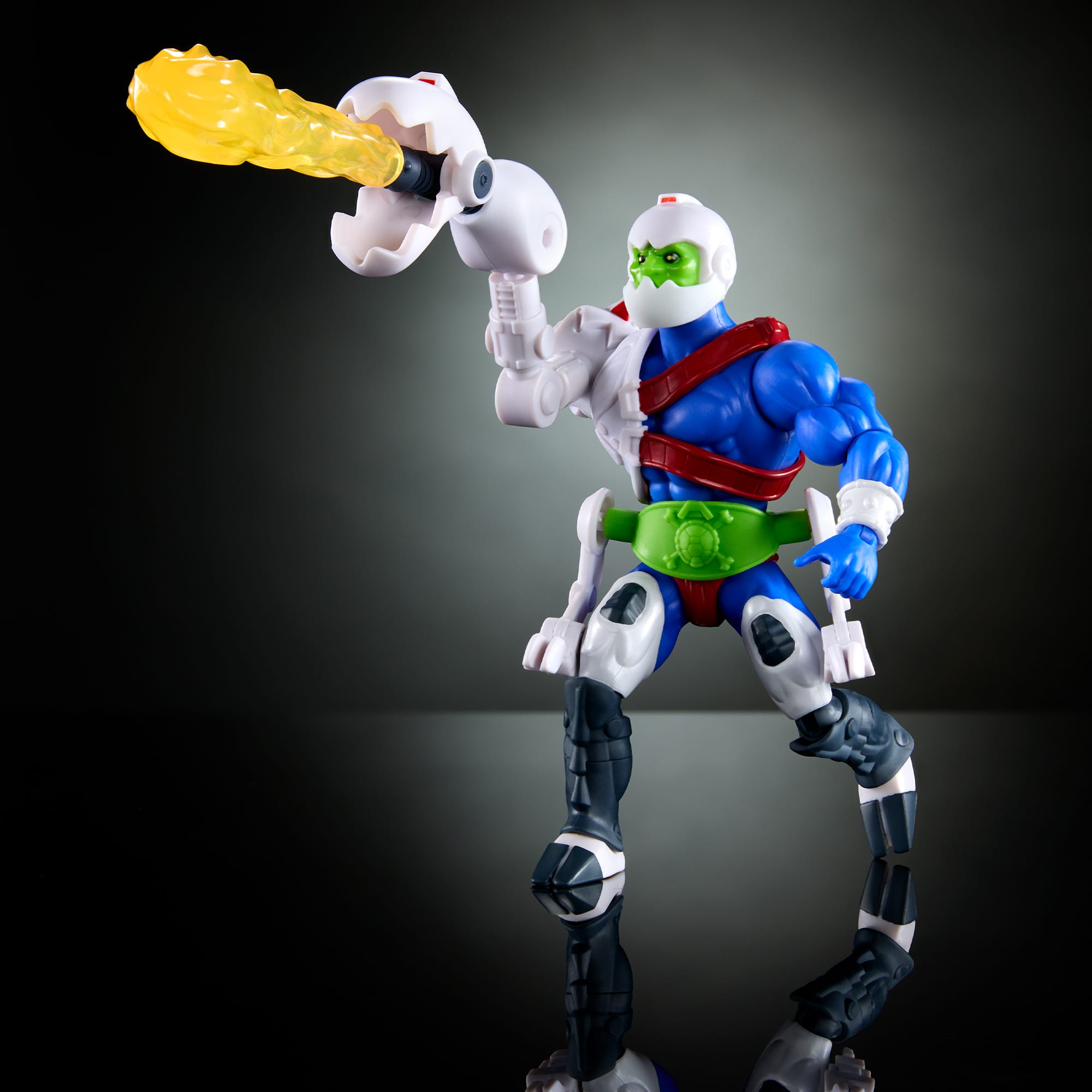This image depicts an intricately designed action figure, reminiscent of a warrior or a character from the Masters of the Universe series. The figure boasts a predominantly muscular blue body, highlighting its humanoid yet potentially alien or robotic nature. The character's face is distinctly green, partially concealed under a white helmet that complements the mechanical aspects of the figure. 

The right arm is noticeably mechanical, equipped with a robotic claw that has an open mouth, from which a yellow plastic flame-like object protrudes, resembling a formidable weapon. The left side, in contrast, displays the action figure's defined musculature, encased in segments of white armor that extend down to its black, two-toed boots. The torso is adorned with a green belt that features a unique emblem—a turtle shell with crossbones behind it. This belt seemingly connects to robotic supports that aid in the mobility of the action figure's legs.

Strapping around the torso and the left arm, a red strap appears to secure the intricate robotic right arm in place, adding to the combat-ready appearance. The figure's attire includes what looks like a championship boxing belt, enhancing its warrior aesthetic. Overall, the combination of vivid colors, mechanical elements, and muscular design makes this action figure a striking blend of strength and advanced technology.